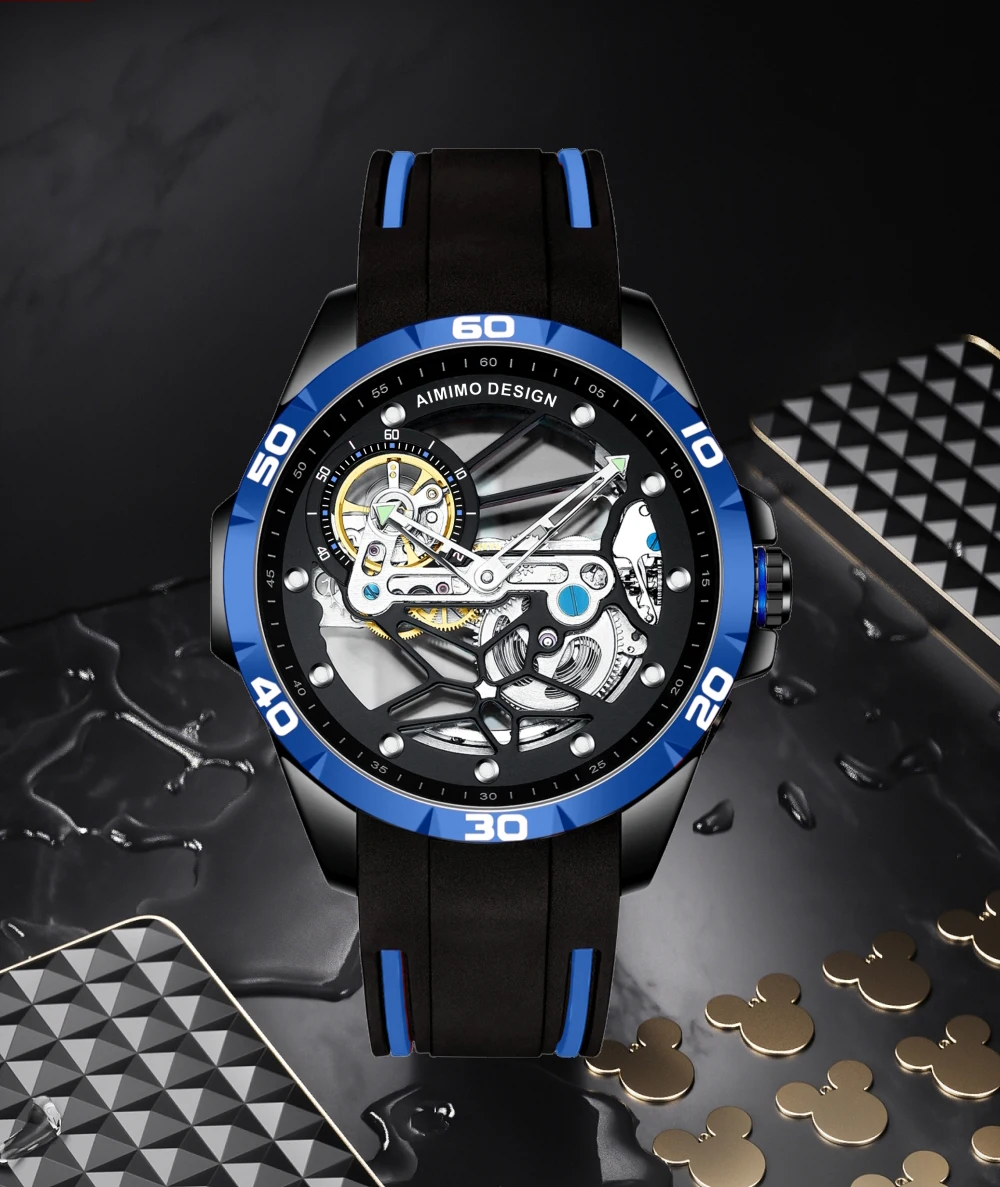The detailed image showcases a close-up, vertically rectangular, full-color photograph of a men's wristwatch. This photograph, which appears to be taken indoors under artificial lighting, reveals a highly unique and intricate design. The watch itself features a round face encased in a blue bezel, with a black inner dial that displays white numbers and letters. Notably, the outer ring of the watch face is marked with large white numbers at 10, 20, 30, 40, 50, and 60, akin to a timer or a specific function watch, rather than a traditional timepiece. The inner ring, showing smaller increments from 5 to 60, subtly hints at its specialized design, along with visible inner mechanics and gears that are exposed, lending a glimpse into the motion of the watch hands. At the top of the inner dial, the text "i-memo design" is prominently displayed in white.

This watch is fastened with a predominantly black wristband featuring blue stripes, lying on a metal table surface that has water splashed on it, resulting in visible wet spots and puddles. Adjacent to the watch, there are several small metal pieces shaped like Mickey Mouse heads, organized neatly in rows in the lower right corner, adding a whimsical element to the arranged scene. The background is a stark black wall and countertop, underscoring the detailed and vibrant elements of the watch and surroundings in this staged setup.